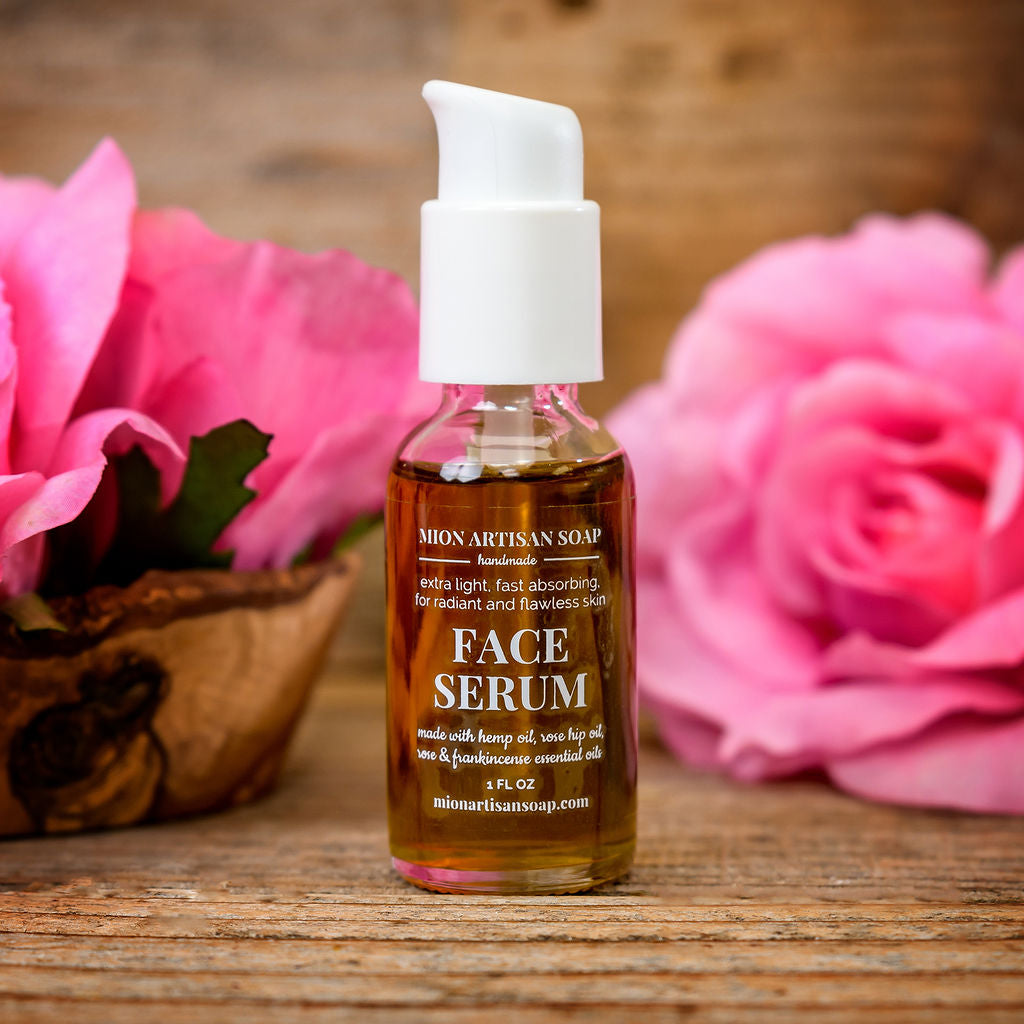This highly detailed promotional image showcases a small, clear glass bottle with a white pump sprayer, filled with a light brown, amber-colored liquid. The bottle prominently displays the brand name "Mion, M-I-O-N, Artisan Soap." In a combination of large and script font, it reads: "HANDMADE, EXTRA LIGHT, FAST ABSORBING FOR RADIANT AND FLAWLESS SKIN." Below that, it states "FACE SERUM" and further details the ingredients, "Made with hemp oil, rose hip oil, rose and frankincense essential oils," along with the volume, "One fluid ounce," and the website, "mionartisansoap.com."

The bottle is set on a wooden surface which makes up both the table and background. To the left, a small burl wood bowl holds a bright pink flower, while to the right, an unfocused large pink rose lies flat on the wooden surface. The background blurs into two pink roses in full bloom, further complementing the serene, nature-inspired aesthetic of the image.